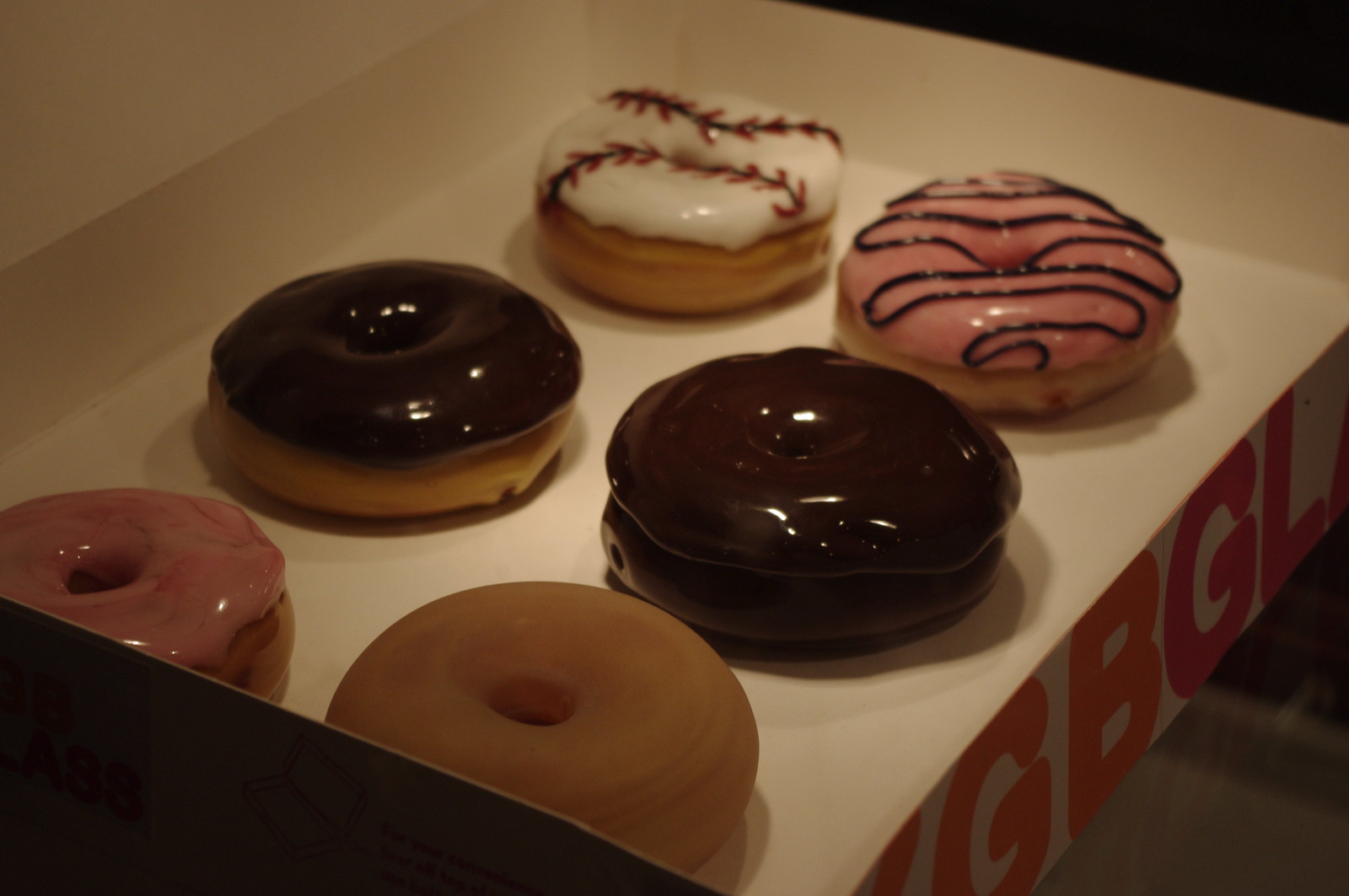The image depicts an open donut box, possibly from Dunkin Donuts, with six glossy donuts arranged inside. The box features orange and pink lettering, although the visible letters, "GBGL," suggest it might not be from Dunkin Donuts. The interior of the box is white. The assortment includes:

1. A plain donut with a light dusting of possible cinnamon.
2. A chocolate frosted donut.
3. A double chocolate donut, fully covered in chocolate glaze.
4. A pink glazed donut with chocolate drizzle.
5. A donut with a white glaze, decorated with red lines resembling baseball stitching.
6. Another pink glazed donut with white drizzle.

The picture, taken from a left-angle view from above, shows the shadows each donut casts, enhancing their glossy appearance. The background includes a white floor, emphasizing the vibrant colors of the donuts.